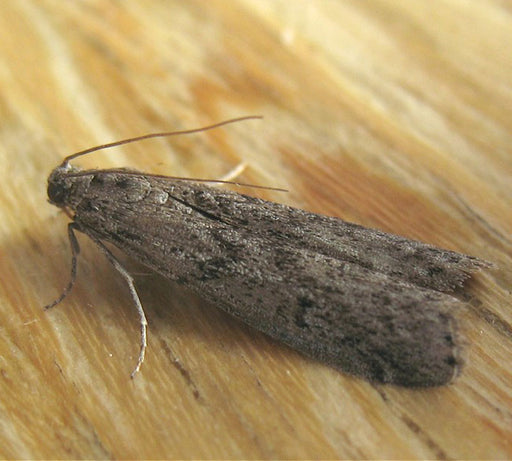The photograph is an extreme close-up of a large, winged insect, identified as a moth. The moth sits centrally on a wooden surface, which appears to be a light brown piece of pine or possibly oak, with visible wood grain. The insect's intricate details are captured in sharp focus, particularly its brownish-gray wings with black spots, giving them a tree bark-like texture. Its two long antennas extend prominently from its small, black head, which is reminiscent of the end of a pin. The moth’s legs are slender and its body is dark brown, almost blending with the wooden surface. The photo's background is blurred, emphasizing the moth's textured back and antennae, suggesting it is resting on the wood. There is no text in the image, and the focus lies squarely on the moth's detailed features, drawing attention to its natural and earthy coloration.